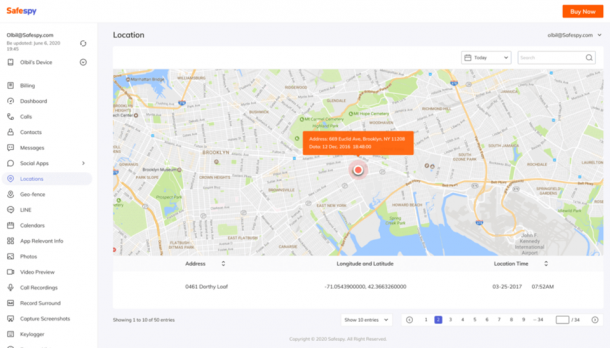The image is a screenshot of a digital interface titled "Safe Spy," displayed in the top left corner. On the left side, there is a vertical menu where the first few options are blurry and unreadable. The readable options listed below include "Billing," "Dashboard," "Calls," "Contacts," "Messages," "Social Apps," and "Locations," with "Locations" being highlighted. Following that are additional options such as another unreadable word, "Line," "Calendars," "App Relevant Info," "Photos," "Video Preview," "Call Recordings," "Record Surround," "Capture Screenshots," and "Keylogger."

To the right of the menu, the interface shows a map of an unidentified area. The map includes text and labels that are too blurry to decipher. Central to this map is an orange circle with an orange dot beneath it. Inside a rectangle on the map, there is some text that is too blurry to read. Below this section, specific details are displayed, including an address, longitude and latitude coordinates, and the location time, with only the location time being legible: "3-25-2017, 7:52 AM."

The screenshot does not contain any photographic elements, people, animals, plants, flowers, trees, or automobiles.